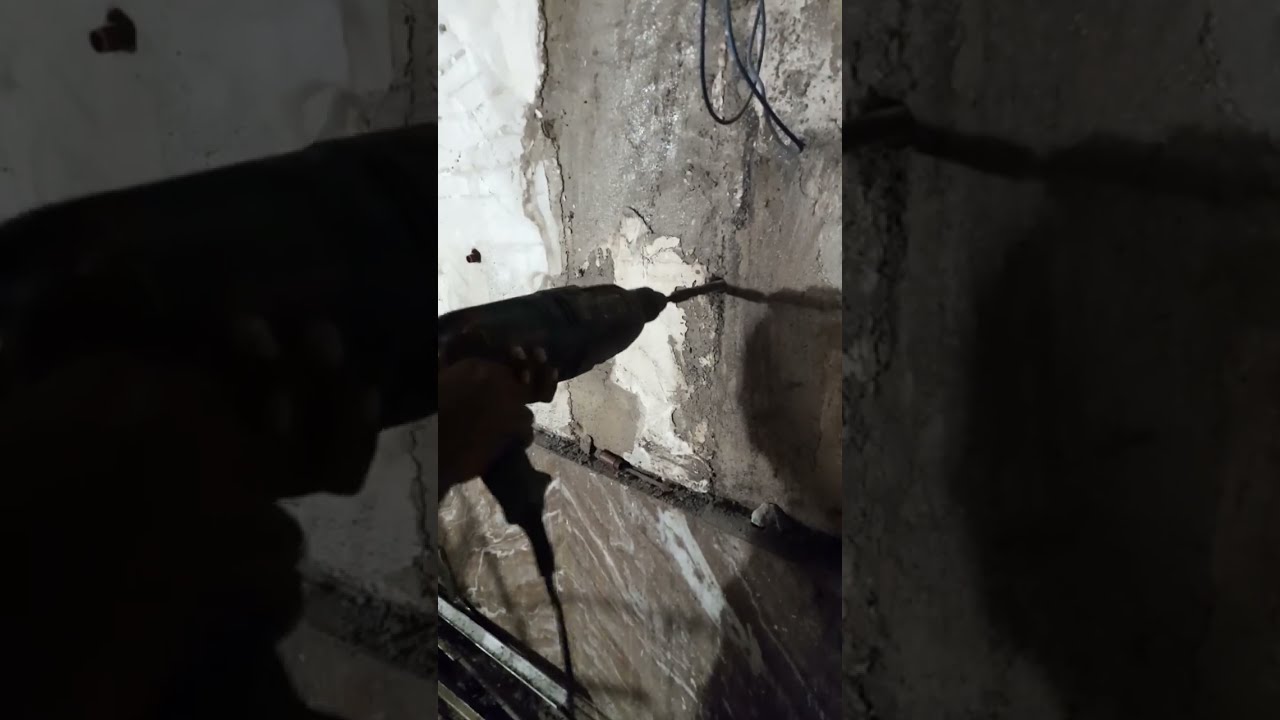The image presents a focused close-up of an electric drill in action, drilling into an unfinished concrete or old gray stone and mortar wall, possibly quite aged. The drill, identifiable by its electric cord hanging from the bottom, extends perpendicularly from the left, and only its silhouette is visible, casting a shadowy outline. A straight, pointy piece, likely the drill bit, protrudes from the drill into the wall. Surrounding this central vertical strip is an expanded, faded, and darkened repetition of the original picture, creating a widescreen aspect ratio effect with mirrored sides. These sides showcase larger, darker versions of the drill and wall, emphasizing the central action. The backdrop includes remnants of old wiring with a bluish tint hanging on the wall. The entire composition gives a detailed, layered view of the drilling process, enhanced by the light subtly entering from the upper left corner, illuminating specific parts of the image.